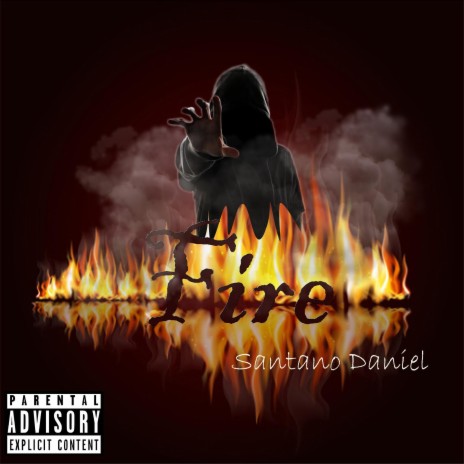The image appears to be an advertisement for a game or possibly a music CD album cover. Dominated by dark hues of black and brown with hints of red, it features a hooded, faceless figure at its center. The figure, cloaked in dark gray or black attire, reaches out towards the viewer with an outstretched hand, exuding an eerie, foreboding presence. Below the figure, flames rise dramatically, casting a vivid reflection as if on water, surrounding the torso with smoke and fiery light.

In the very center of the image, the word "FIRE" is prominently displayed in large, dark brown or maroon letters, styled in a creepy, unsettling font. Beneath this title, in much smaller, thin white letters, is the apparent creator's name, "Santano Daniel." The bottom left corner of the image contains a Parental Advisory Explicit Content warning, set within a small white box.